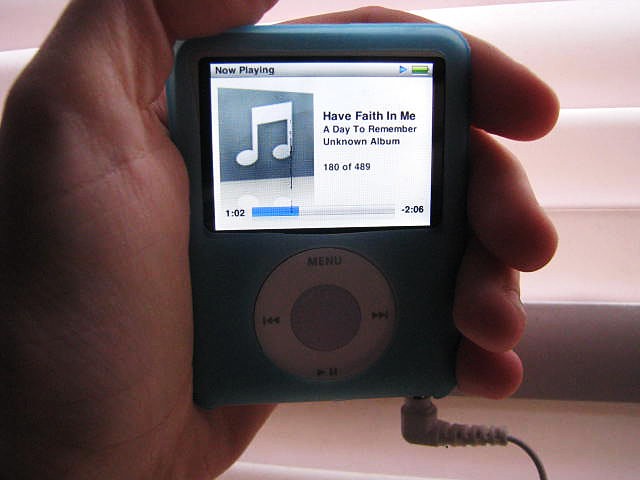In this detailed landscape-oriented color photograph, the central focus is a person's hand emerging from the left side, holding an iPod centrally positioned in the image. The iPod's screen is illuminated, displaying the text "Now Playing" across the top, followed sequentially by "Have Faith in Me", "A Day to Remember", and "Unknown Album". Additionally, it shows "180 of 489" and indicates there is one minute and two seconds left on the current song. A blue progress bar is visible at the bottom of the iPod screen. An electrical cord extends from the bottom of the device, suggesting it is plugged into a power outlet. The background features a partially open white blind, with visible lines suggesting it is indoors during daytime. The photograph emphasizes the combination of white, tan, blue, dark blue, and gray colors in its composition.